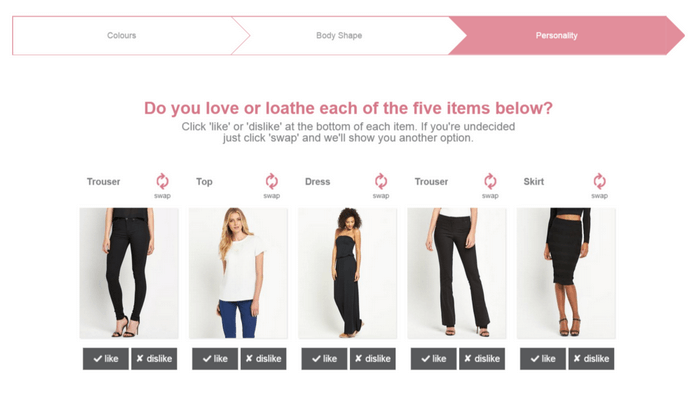The image showcases a webpage with a clean white background designed for user interaction to express preferences about clothing items. At the very top of the page, the categories "Colors," "Body Shape," and "Personality" are prominently displayed, suggesting a focus on personalized fashion recommendations. Beneath these headings, in striking pink or red text, a prompt asks users, "Do you love or loathe each of the five items below? Click like or dislike at the bottom of each item. If you're undecided just click swap and we'll show you another option."

The main section of the page features five clothing items arranged side by side, each paired with an image and descriptive texts:

1. **First Item**:
   - Label: "Trouser"
   - Image: A woman wearing black trousers.

2. **Second Item**:
   - Label: "Top"
   - Image: A blonde woman in a white t-shirt.

3. **Third Item**:
   - Label: "Dress"
   - Image: A woman adorned in a full-length black dress.

4. **Fourth Item**:
   - Label: "Trouser"
   - Image: Another depiction of a woman in black trousers.

5. **Fifth Item**:
   - Label: "Skirt"
   - Image: A woman wearing a black skirt.

Below each image, there are interactive buttons labeled "Like" with a check mark and "Dislike" with an X. At the current stage, none of these options have been selected. Additionally, each clothing item includes a "Swap" option, indicated by a circular arrow, allowing users to choose a different option if they are undecided.